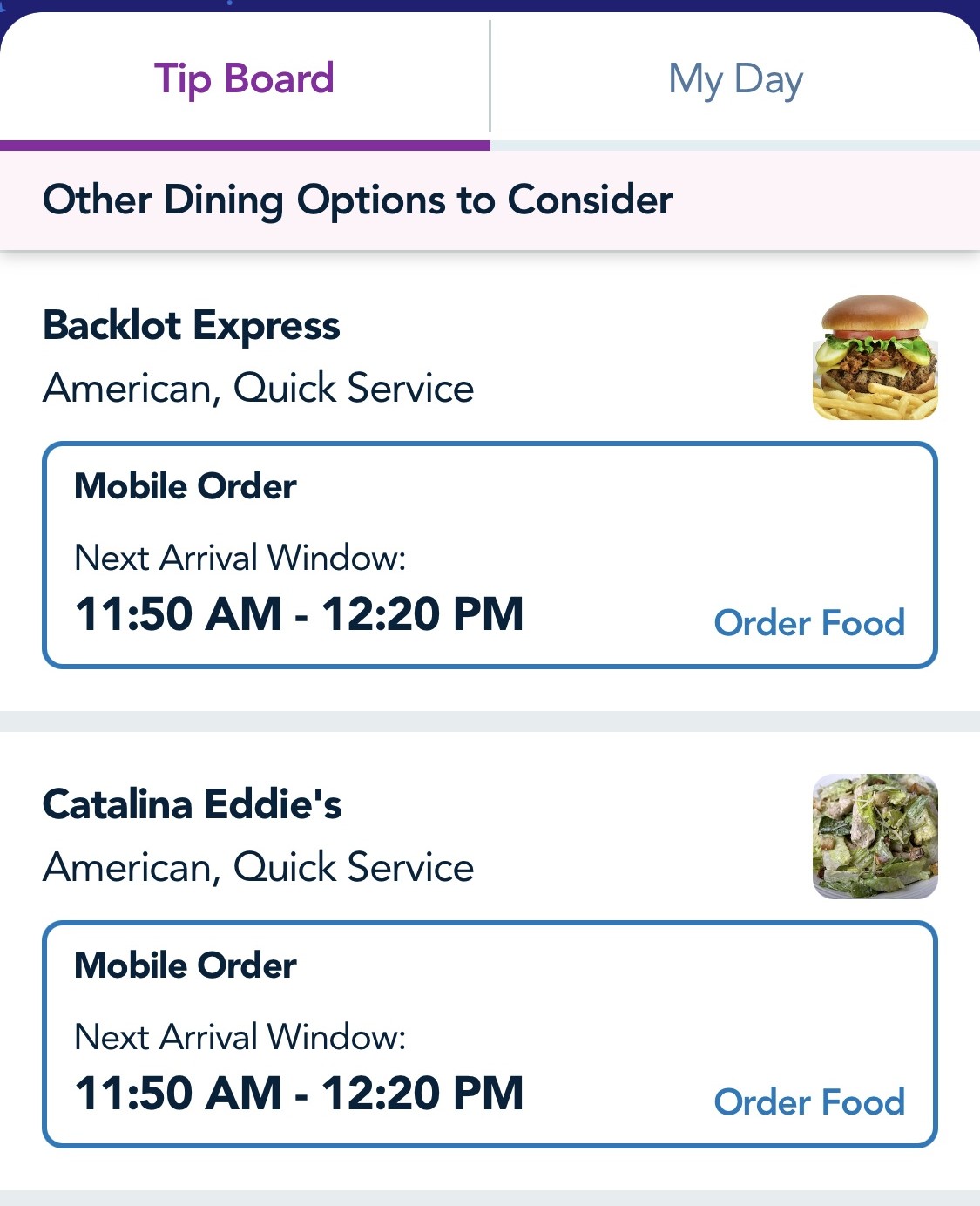This screenshot features a detailed view of a menu from an application titled "Tip Board." The menu splits into two sections, "Tip Board" and "My Day," highlighted by a purple underline. Below it, there's a section suggesting "Other Dining Options to Consider," which lists different dining venues and their offerings.

First on the list is "Backlot Express," described as an American common service restaurant. The menu includes items such as hamburgers garnished with lettuce, tomatoes, pickles, cheese, and served with french fries. The option to place a mobile order is prominently displayed, with the pickup window specified as 11:50 AM to 12:20 PM. The "Order Food" option is highlighted in blue.

Next, "Catalina Eddie's," another American common service spot, follows under a grey bar. The menu highlights a salad as a key offering. Similar to Backlot Express, the mobile order service is available from 11:50 AM to 12:20 PM, with the "Order Food" option also highlighted in blue.

All text in the menu is rendered in black, with distinctive blue text for actionable items like placing an order.